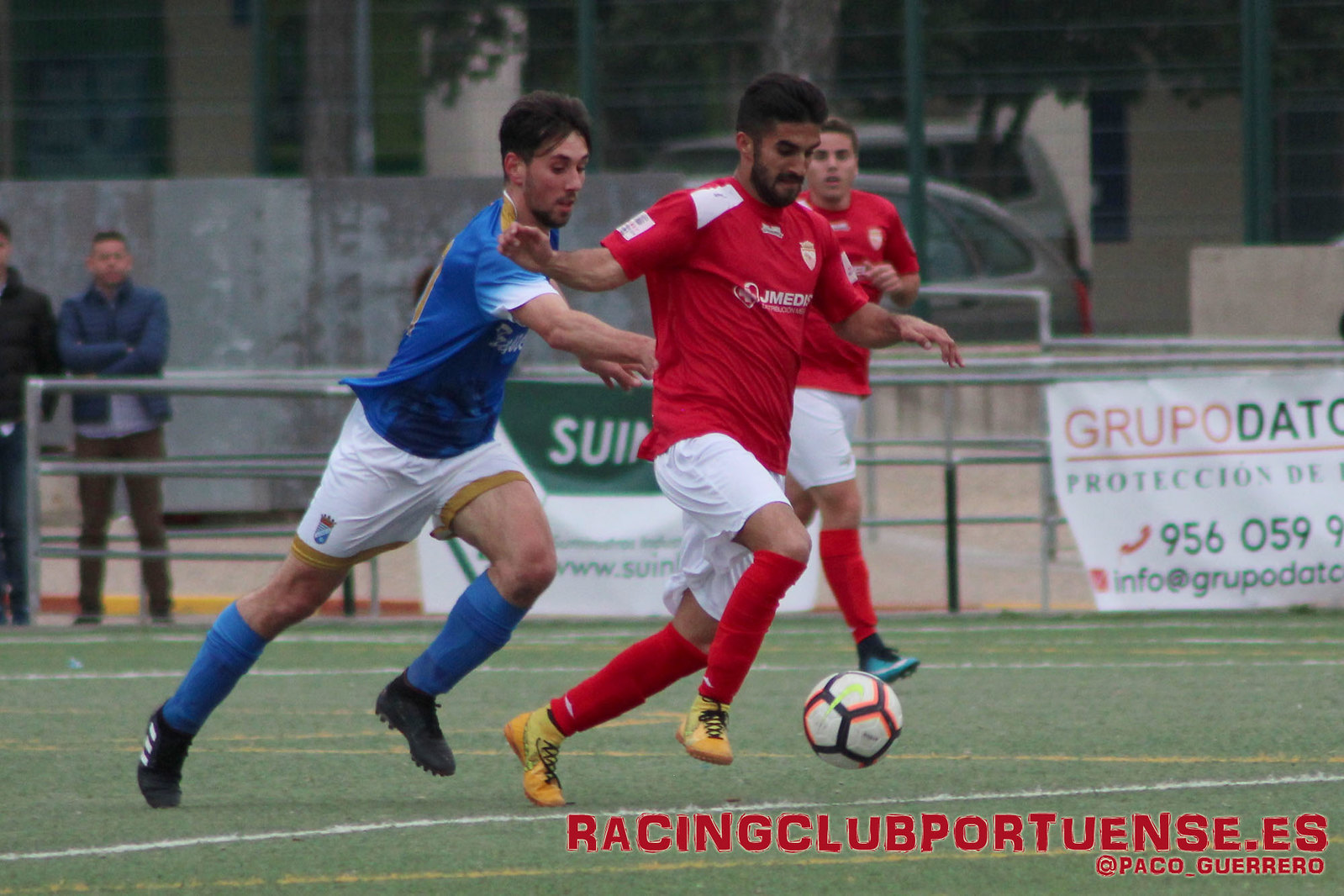This vibrant color photograph captures an intense moment in an outdoor soccer game. Three young men dominate the scene, all engaged in a high-energy battle for the soccer ball on a well-maintained field. The focal point is on two players in the foreground: one in a red jersey with white shorts and red socks, wearing yellow shoes, and another in a blue jersey with white shorts and blue socks, sporting black shoes. The player in red is trying to kick the ball away from the player in blue, who is closely shadowing him, making a determined attempt to take control. Both players are mid-action, with one foot planted on the ground and the other in mid-air, embodying the dynamic intensity of the game. A third player in a red jersey and white shorts can be seen in the background, running to support his teammate. Surrounding the field are concrete walls and green fences designed to keep the ball in play. On the periphery, a group of coaches dressed in black and white suits watch the game attentively. The perimeter fence is adorned with numerous advertisements, including "Grupo Dei" and "Proteccion." A web address, "RacingClubPortuense.es," alongside the handle "@PacoGuerrero," is visible at the bottom right corner of the image, serving as a watermark for this action-packed shot.